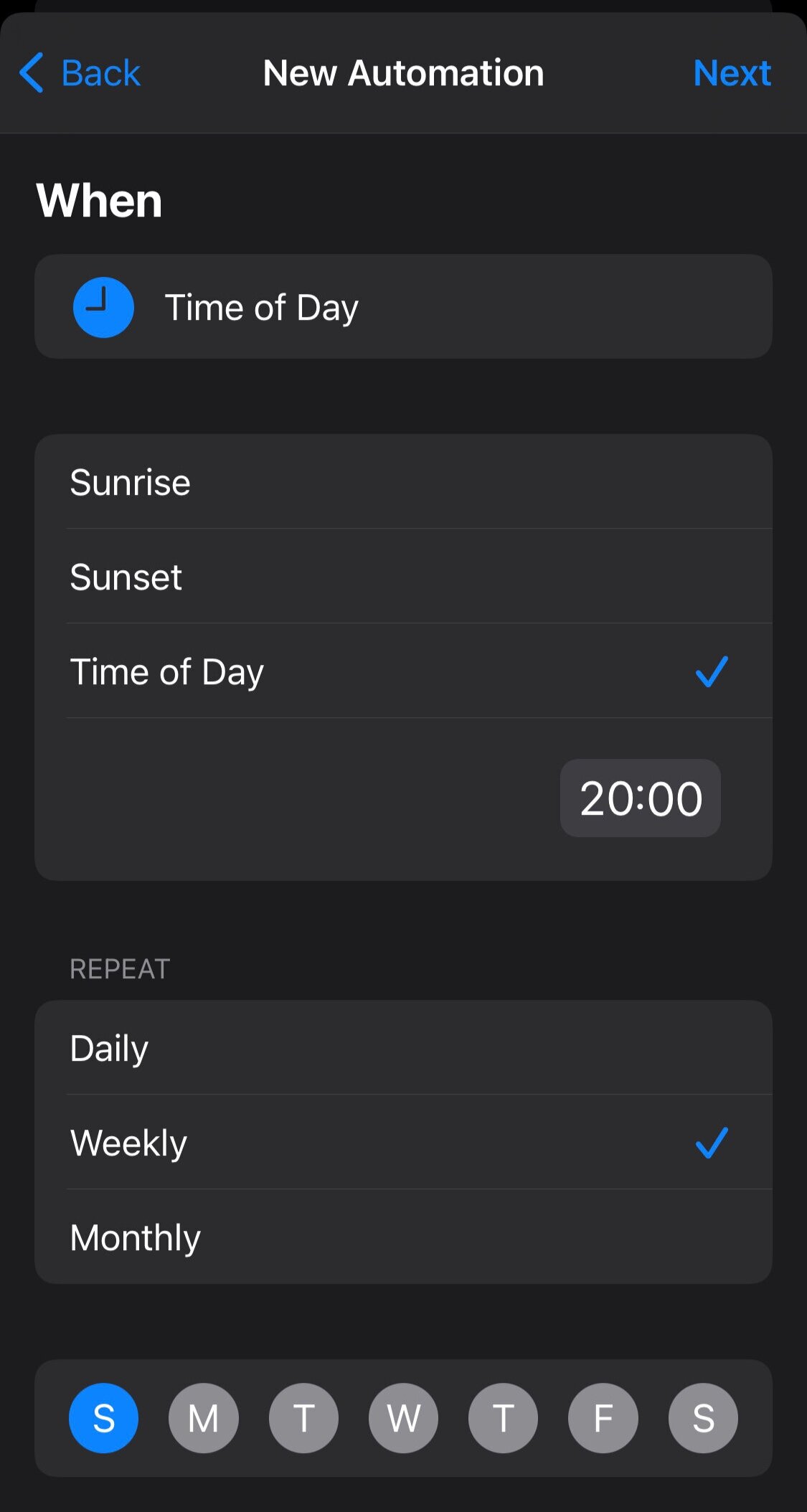This screenshot, captured on a cell phone, displays a user interface with a black background. At the top-left corner is a blue "Back" button accompanied by a leftward-facing blue arrow. On the opposite side at the top-right corner is a blue "Next" button.

Centrally positioned in white text, the screen reads "New Automation." Directly beneath, in white letters, the text "When" is displayed. Under this heading, the text "Time of Day" appears next to a blue clock icon indicating the minute and hour hands.

Further down are three options listed in white text: "Sunrise," "Sunset," and "Time of Day." A blue checkmark is situated beside "Time of Day," which is followed by "20:00," indicating 8:00 PM in military time.

Below this, options for "Repeat" frequencies are listed: "Daily," "Weekly," and "Monthly," again in white text. The "Weekly" option has a blue checkmark beside it. Underneath these options, there are seven circles representing the days of the week: Sunday, Monday, Tuesday, Wednesday, Thursday, Friday, and Saturday. Among these, only the circle for Sunday is blue, implying it is selected, while all other circles remain gray.

This setup suggests that the user is configuring a new automation, likely an alarm, set to activate at 8:00 PM every Sunday.